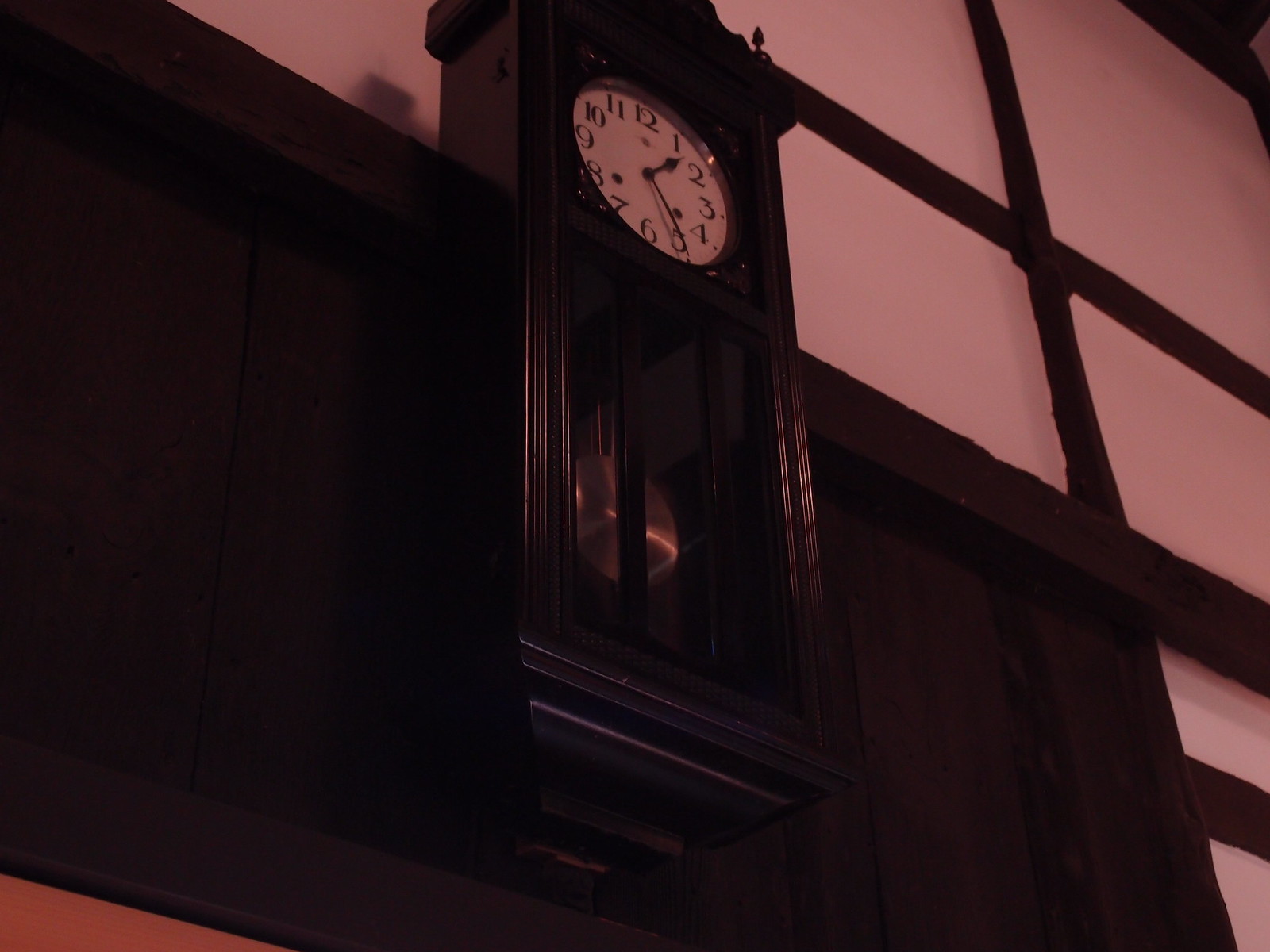The photograph captures an indoor setting, showcasing a large, polished, dark brown wooden grandfather clock mounted on a light-colored wall. The wall, possibly light pink due to the lighting, features dark brown wooden trim. The wall also has a distinctive brown section. The clock, reminiscent of a Tudor style, has an exposed wood and a glass case that extends from the middle to the bottom, revealing a shiny gold or silver pendulum. The clock face is white, though it appears light pink under the lighting, and is adorned with black numbers from 1 to 12. The black metal hands of the clock indicate the time as approximately 1:25. Above the clock, the wall is trimmed with dark timber beams, adding to the room's classic aesthetic.